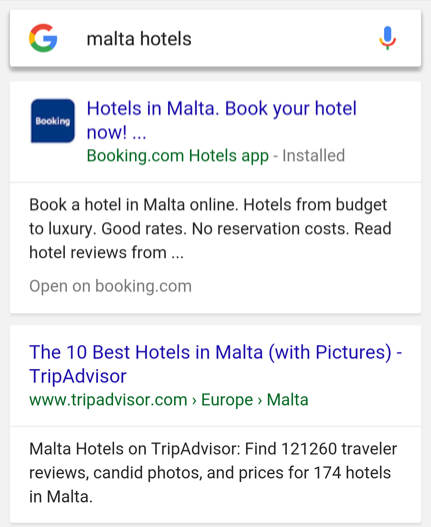The image depicts a Google search results screen with a focus on Malta hotels. At the top, the search bar contains the query "Malta hotels". To the left of the search bar, there is the iconic multicolored Google "G" logo in red, yellow, green, and blue. On the right, there's a blue microphone icon for voice search.

The first search result appears in blue text and reads "Hotels in Malta – Book your hotel now". Directly beneath it, "booking.com/hotels" is listed in green, identifying the website. The brief description below provides more details: "Book a hotel in Malta online. Hotels from budget to luxury, good rates, no reservation costs, read hotel reviews from… Open in booking.com".

Further down, the second result is from TripAdvisor, labeled "The 10 Best Hotels in Malta (with Pictures)" in blue text. Below this, the URL is displayed as "tripadvisor.com/europe-malta". The description summarizes the content as "Malta hotels on TripAdvisor. Find 121,260 traveler reviews, candid photos, and prices for 174 hotels in Malta."

The entire content is set against a clean, white background, presenting a typical view of a Google search results page.